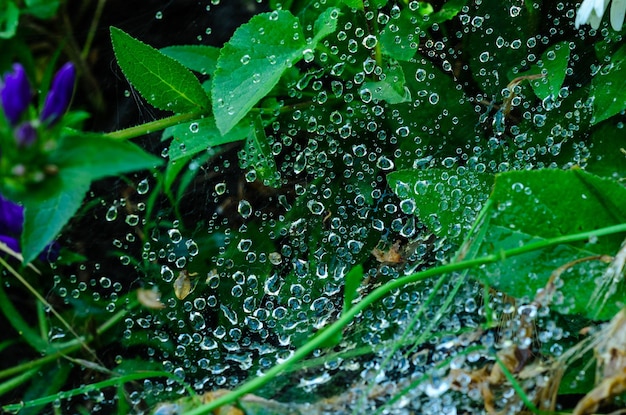This close-up image showcases vibrant green leaves, likely ivy, adorned with numerous, crystal-clear water droplets of varying sizes. These droplets, a result of either gentle rainfall or morning dew, are delicately supported by an implied, nearly invisible spider web. On the leftmost edge of the photo, three brilliantly colored bluish-violet tubular buds emerge amidst the foliage, adding a striking contrast. In the background, more leaves fill the scene, while at the bottom center, a green stem extends towards the right. Small brown-yellow leaves peek out from the lower right corner, suggesting the plants are on the ground. The overall impression is one of fresh vitality and serene beauty in a natural setting.